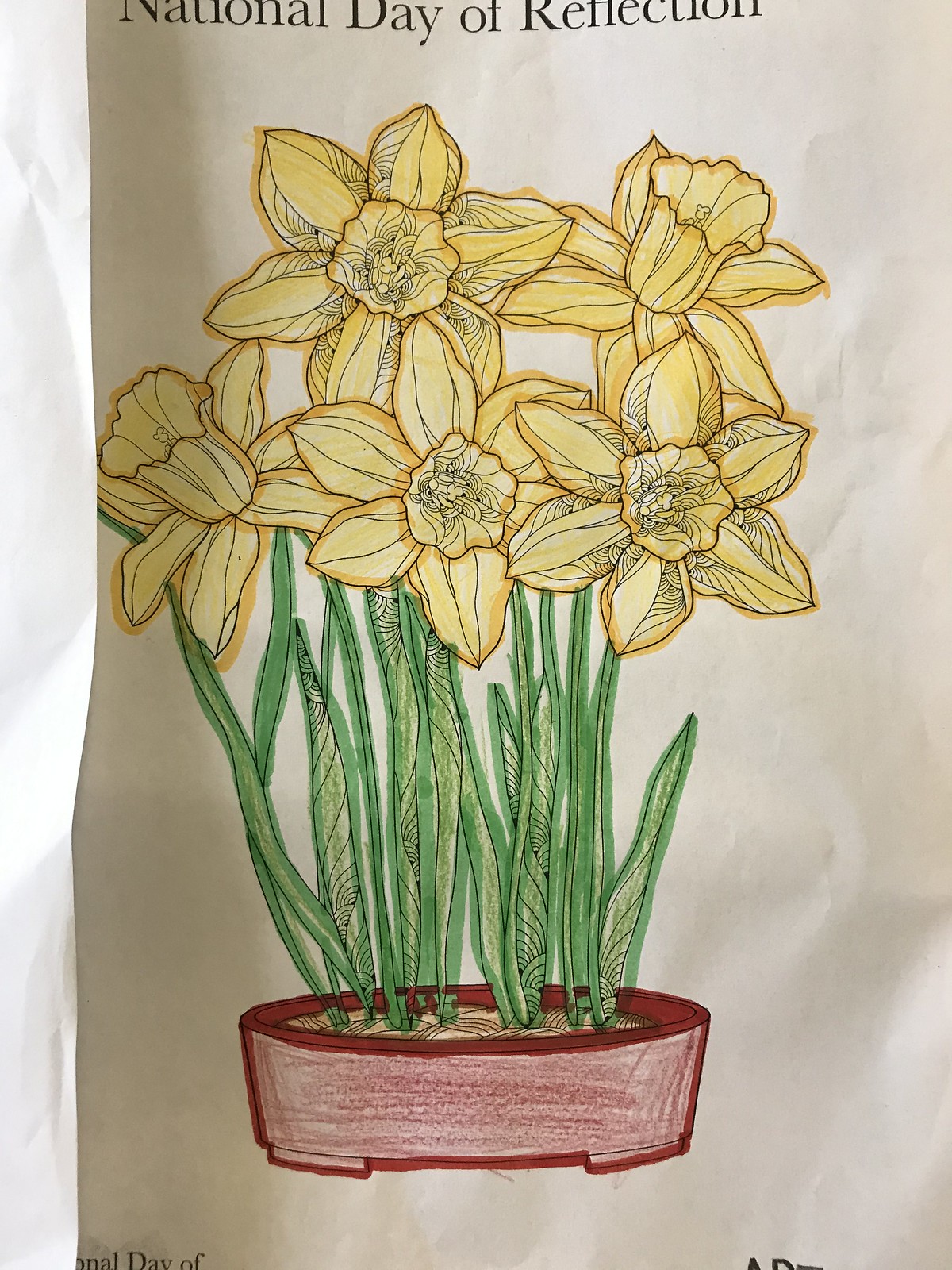The image is a roughly vertical piece of crumpled, light gray paper, possibly aged from what was once white. At the top, partially cut off, in black type text, it reads "National Day of Reflection." The central focus of the image is a pre-printed drawing of a low, circular pot containing five daffodils, which has been colored in by hand. The pot, resembling an ashtray, is short, red, and filled with brown soil, featuring low-profile legs. From it emerge long green stems adorned with long, narrow leaves. The daffodils, each with six petals, are inconsistently colored with yellow and shades of gold markers. The overall coloring appears somewhat unrefined, suggesting it might have been completed by a child. The paper's worn texture adds to the piece's casual, homemade charm, making it a fitting decoration for a day of national reflection.